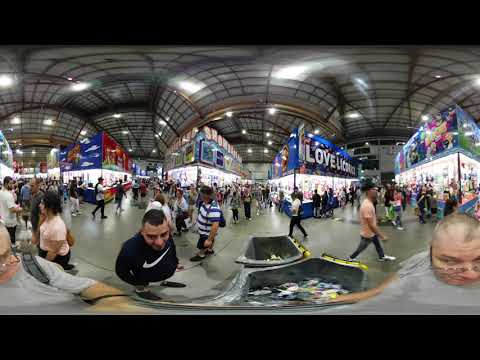The image portrays a bustling shopping mall or marketplace seen through a fisheye lens, which distorts the scene into multiple rounded segments. Centrally, the area is crowded with people milling about, engaging in commerce and conversations. Visible are four storefronts, prominently featuring a candy store with a sign that reads "I Love Licorice". In the foreground, several individuals stand out: a dark-haired man in a Nike sweater, a bald man in a grey shirt and glasses, and a woman in a pink shirt with a purse over her right arm. The environment features industrial, shiny, grey concrete floors and a high ceiling supported by black grid and beam structures. Lighting fixtures are mounted on the beams, providing illumination across the bustling, vibrant floor space.